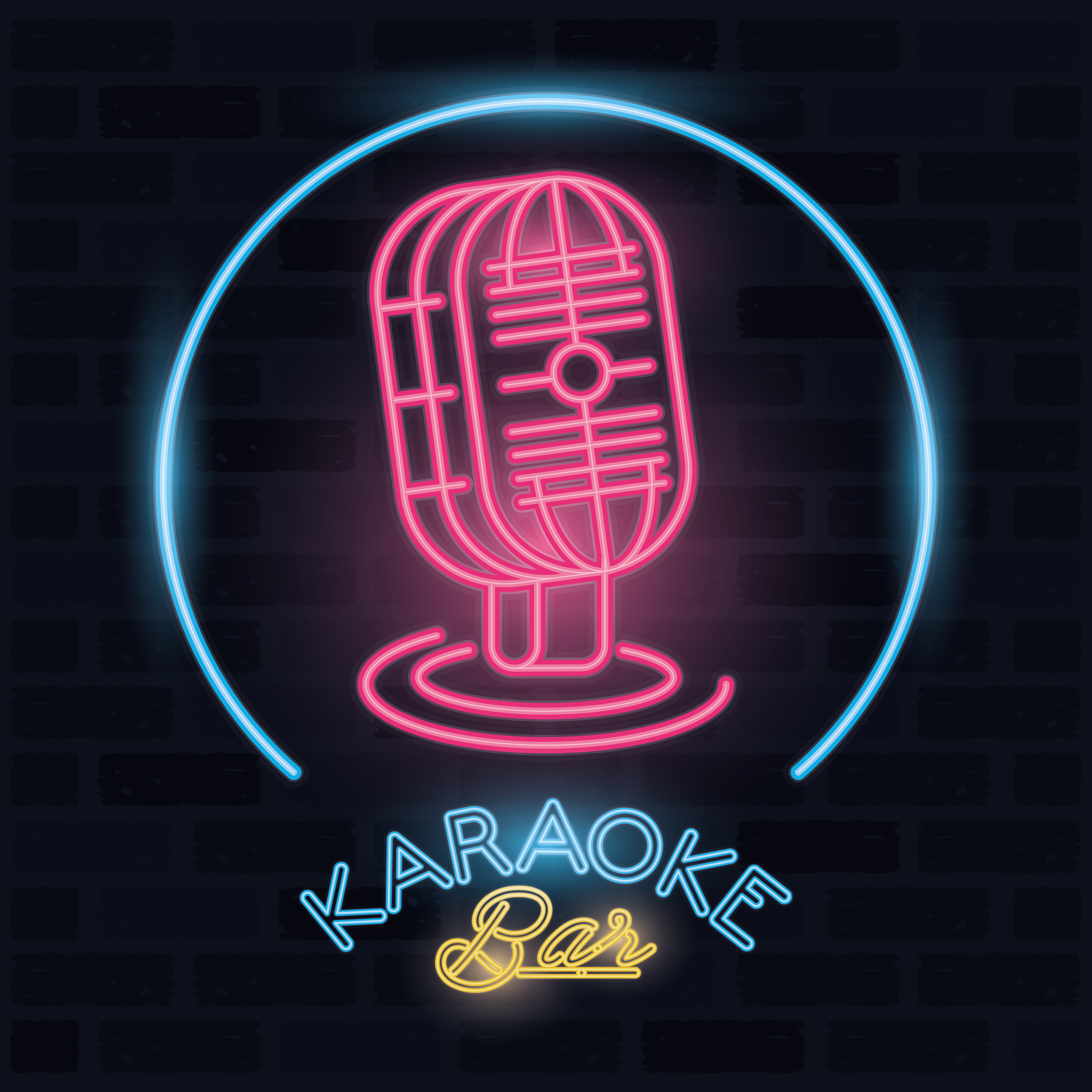The image is a vibrant and creative advertisement for a karaoke bar, set against a predominantly black background. Faintly visible through the dark backdrop is a textured brick wall, adding a subtle touch of depth. Dominating the foreground is a striking illustration of an old-fashioned microphone in pink neon, reminiscent of those seen in early 20th-century films. This microphone is encircled by a nearly complete ring of blue neon light, which creates a vivid contrast. Below the microphone, in capitalized blue neon letters, is the word "KARAOKE," followed by the word "bar" in a yellow, handwritten neon style. This clever graphic design, likely produced using computer software, uses different fonts to emphasize its themes and adds a lively touch to the minimalistic scene, making the neon lights pop against the dark, brick-adorned background.